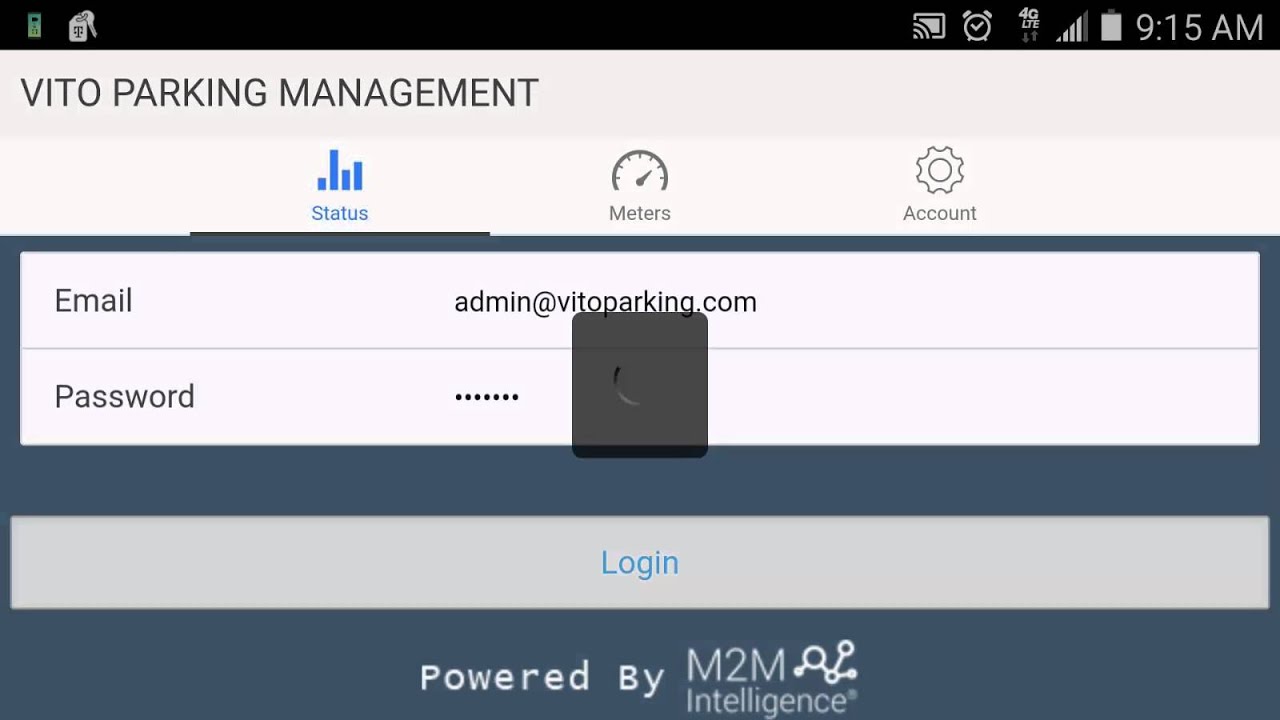The image shows a screenshot of a smartphone, captured at 9:15 a.m. The phone is connected to a 4G network and the battery icon shows a nearly full charge. The screen displays a login page for "Veto Parking Management." 

At the top of the page, there are three tabs labeled "Status," "Meters," and "Account," with the "Status" tab highlighted in blue, while the other two are gray. The central part of the screen displays fields for an email address and a password (obscured by dots for privacy), with a gray "Login" button below them. The text "Login" is highlighted in blue.

Below the login button, the text "Powered by M2M Intelligence" is displayed in white against a blue-gray background, which extends as a border around the email and password fields. The background of the email and password fields is white with black text.

In the middle of the screen, there's a gray circular overlay, indicating that the app is processing the login attempt. The curved gray line within the overlay suggests a loading or progress indicator.

Overall, the screenshot appears to capture the moment someone is attempting to log in to check their parking status or manage their parking account.